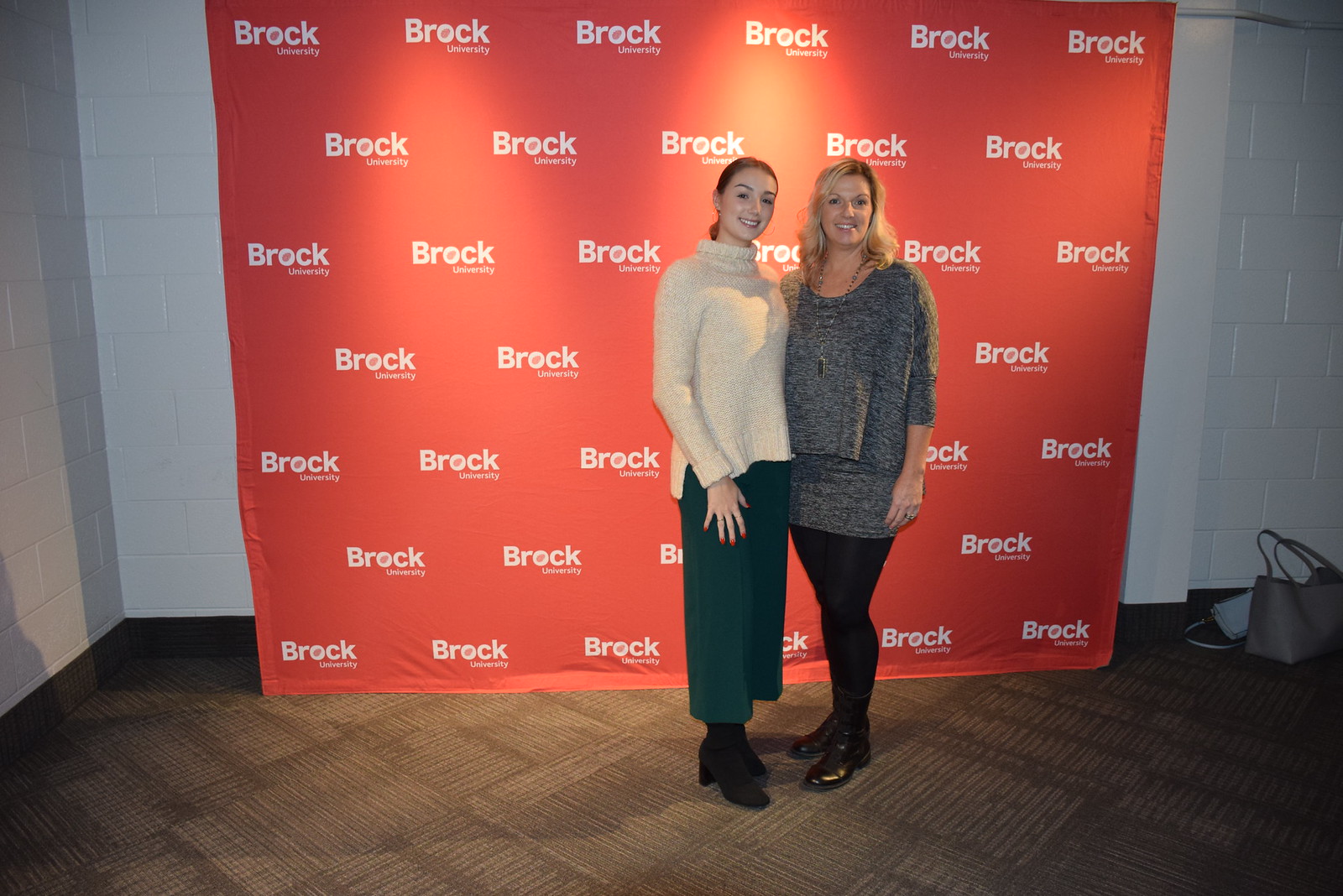In this photo, two women are standing together in front of an orange banner that prominently features the repeated logo and text of "Brock University," against a backdrop of white-painted cinderblock walls. The women are positioned slightly to the right of the center of the image, standing on a brown textured carpet. 

The woman on the left is wearing a white turtleneck sweater paired with a dark green skirt that reaches down to her ankles. She is also wearing black high-heeled boots. Her nails are painted red, and she has red hair tied into a ponytail. Her right arm appears to be around the woman next to her.

The woman on the right is dressed in a gray top and matching gray skirt, complemented by black leggings and black boots. She has blonde hair and is wearing a necklace and a ring on one of her fingers. To the far right of the image, there are two bags placed against the wall—a larger brown bag and a smaller white one—seemingly set aside to keep the foreground clear for the photo.